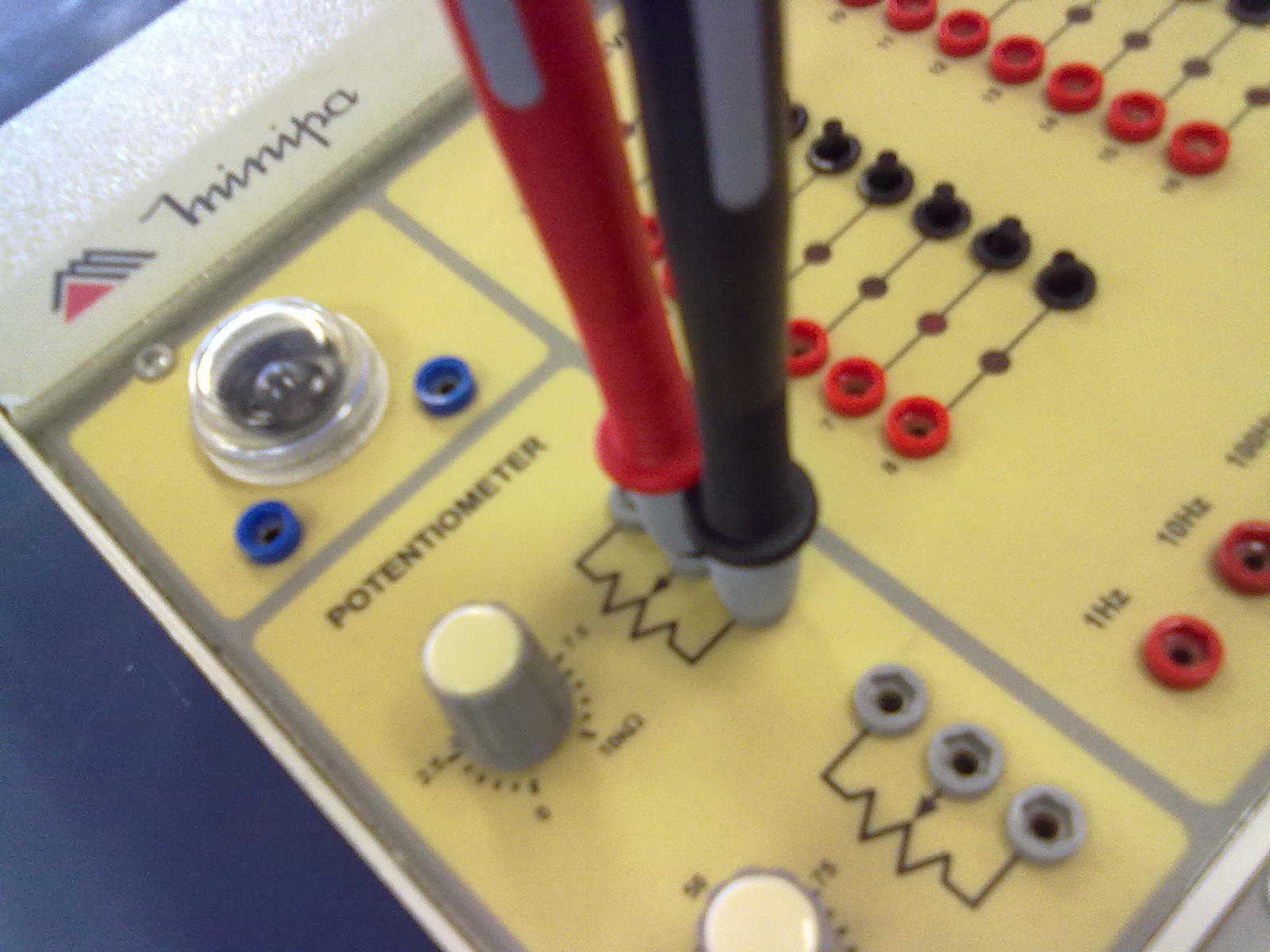The image depicts a detailed view of a yellow electrical board labeled "potentiometer" on the left, featuring a prominently positioned knob. The board includes various electronic inputs and circuit drawings. Towards the bottom, there are three jacks labeled "1 Hertz," "10 Hertz," and "100 Hertz," respectively. The top right section showcases multiple red and black circles; the black ones have protruding pins while the red ones are recessed. Additionally, the board displays red, gray, and black circles, indicating connection points. A somewhat unclear name, which appears to be written in cursive, is present at the top of the board, potentially reading "i n i n i p a." This setup suggests that the board might be used for educational or practice purposes in electronics.